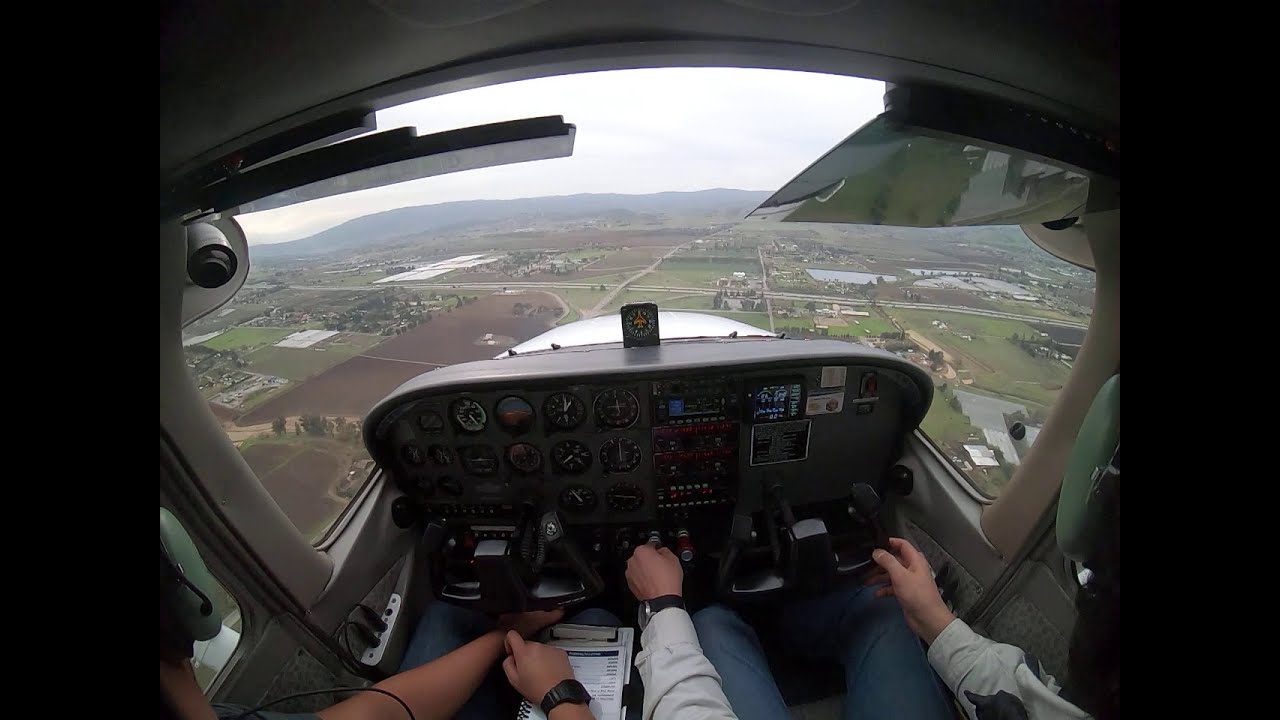This photograph captures an intimate scene inside the cockpit of a small aircraft, possibly a helicopter or a light airplane. The cockpit is filled with various controls, dials, and gauges although no specific text can be read from them. Two individuals are seated closely together due to the cramped nature of the space. The person on the right, distinguishable by their watch, is actively engaged with the aircraft's controls, holding the steering wheel with one hand and pressing a dial with the other. The person on the left, also wearing a watch but on the opposite wrist, is holding a manual or a set of papers, likely indicating a training or instructional session. Both individuals appear to be immersed in their tasks, and they are wearing headphones, possibly for communication purposes.

Outside the cockpit, the scenery below unfolds into a patchwork of green and brown fields interspersed with roads and occasional buildings, suggesting a rural or countryside setting. Despite not being very high up, the landscape still appears somewhat distant and small. The sky above is mostly overcast with a hint of blue, and in the far distance, a line of mountains stretches across the horizon, adding depth to the scene. The entire photograph, roughly 8 inches wide and 5 inches tall, captures not only the intricate details of the cockpit but also the expansive, yet hazy, landscape beyond.